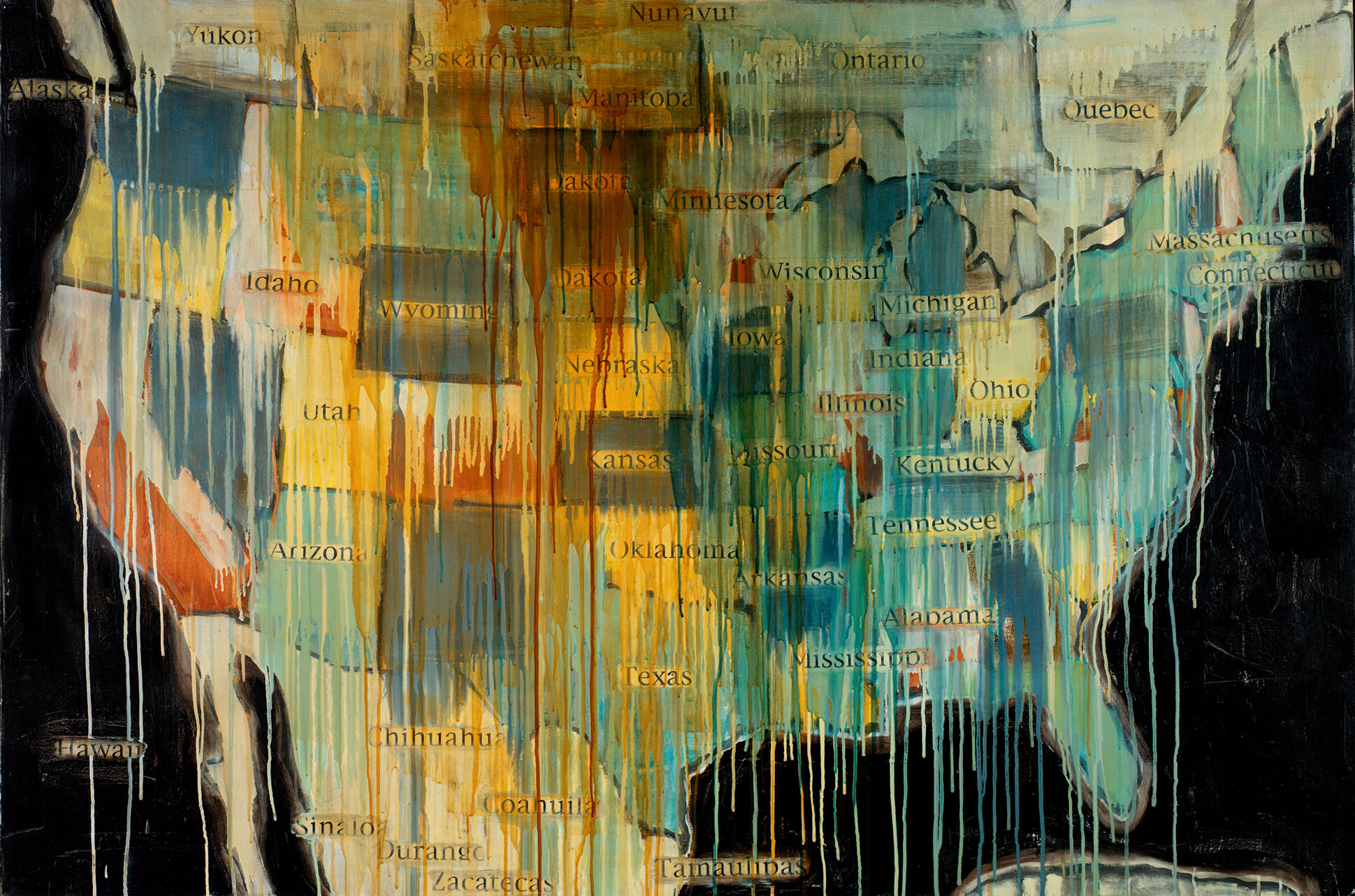This vibrant and evocative painting captures a dripping, dreamlike representation of North America. The core of the piece is a detailed map of the United States, with each state delineated and filled with a kaleidoscope of colors, including shades of blue, red, yellow, light blue, off-white, and gray. The colors are heavily blended and streaked, creating a fluid, melting effect across the entire painting. The background is a deep black, enhancing the vividness of the dripped paint.

Some of the states are labeled in black, including notable mentions like Minnesota, Wisconsin, Iowa, Illinois, Oklahoma, Kansas, Massachusetts, and Connecticut, though not every state name is visible due to the paint's coverage. Along the top of the artwork, various provinces of Canada such as Yukon, Saskatchewan, Ontario, and Quebec are also displayed, seamlessly transitioning from the U.S. border. Moreover, parts of Mexico, including regions like Chihuahua, Sinaloa, and Durango, are seen along the bottom left, showing their connection to the southern U.S. states like California, Arizona, and Texas. 

The entire artwork has an appearance as if thin or watered-down paint was allowed to run from top to bottom, creating a vertical cascade of colors that blurs and blends state borders and names, giving the map a surreal, almost ethereal quality. This warped, dripping appearance evokes a sense of motion and fluidity, transforming a standard map into a mesmerizing piece of abstract art.